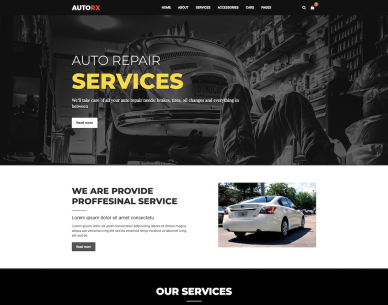This is a detailed caption for the imagery provided:

---

The image is a screenshot depicting either an advertisement or the homepage of a company’s website dedicated to car repair services. At the top of the page, a banner features the company name "Auto RX." The word "Auto" is displayed in white, while "RX" is in red, both in all capital letters. The top banner also includes navigation options such as "Homepage" and "Email." However, due to the image's clarity, some finer text within the banner remains unreadable.

Below the banner, the focal point of the page is a prominent image of a car repair scene. The vehicle in the image is an older model Volkswagen, and a mechanic is seen working underneath the car. This visual is accompanied by text that reads, "Auto Repair Services," followed by an incomplete message likely stating, "We will take care of your car." Viewers are prompted to read more by clicking on the relevant link.

Further down, there's a statement highlighting the professional nature of the services offered: "We provide professional service." At the very bottom, a black bar with white text appears to offer navigation to detailed information about the services available, presumably labelled "Our Services." This section is intended to guide users seeking more specific details on what the company offers.

The overall design suggests that the page serves as either a targeted ad or the homepage for a car repair service company, emphasizing professionalism and customer care through its visual and textual elements.

---